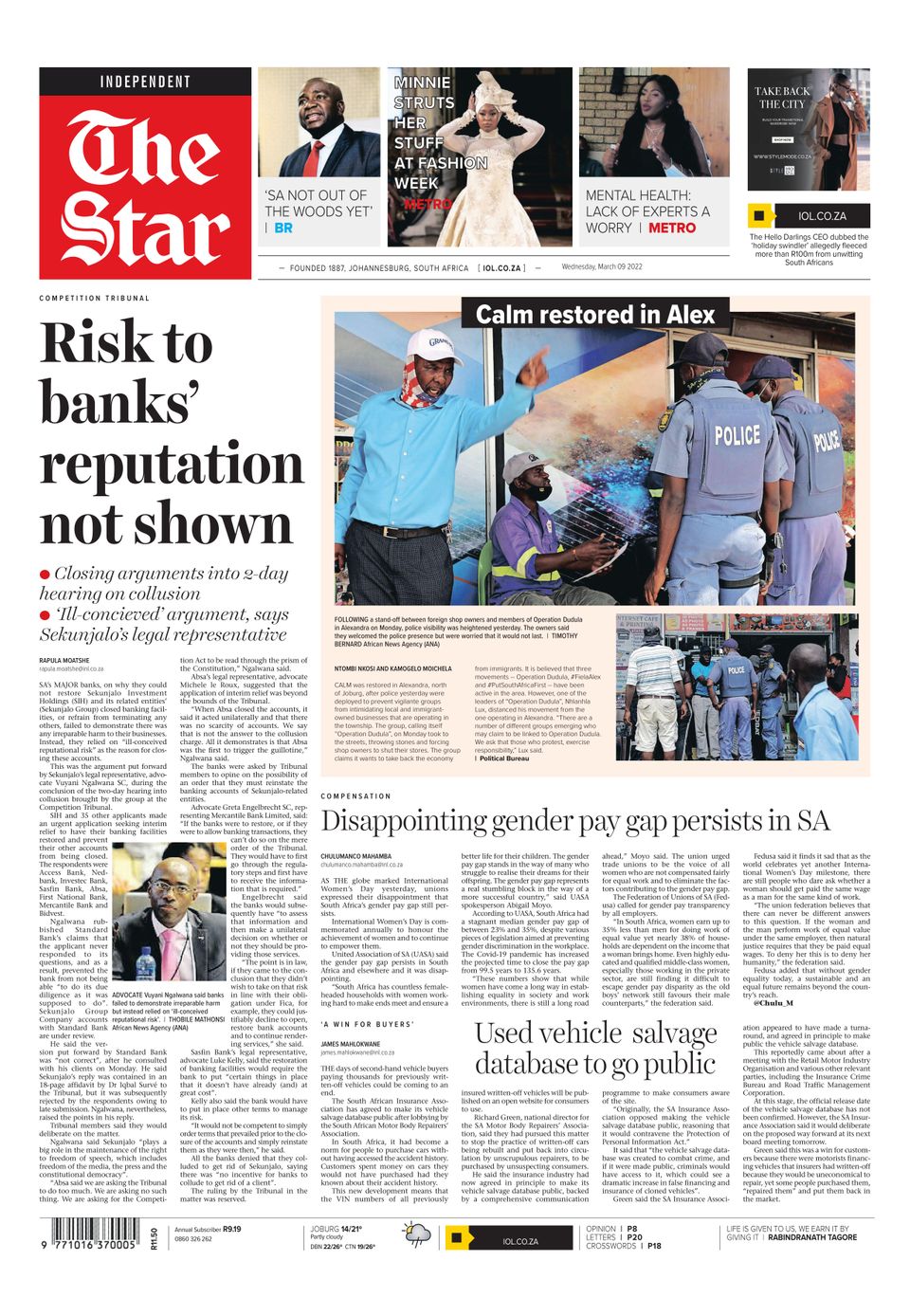The front page of the newspaper features a rich array of articles and images, organized to capture immediate interest. 

At the very top left corner, the masthead consists of a distinct logo: a thin black border encloses a red box, within which the word "The Star" is elegantly scripted in a fancy calligraphy font. Adjacent to it, in a white text against a black background, the word "Independent" is positioned prominently.

To the right of the masthead, there are four smaller boxes, each containing headlines and images. The first box features an image of a bald Black man in a suit with a red tie, accompanied by the headline: "S.A. not out of the woods yet." The second box shows a woman dressed in an elegant white dress and headpiece under the text: "Many threats her stuff at Fashion Week," tagged with a red "Metro" label underneath. The third box contains an image of a Black woman with long black hair engaged in conversation, accompanied by the headline: "Mental health, lack of experts, a worry," also tagged with "Metro" to the right. The fourth box appears to be an advertisement, showing a person wearing a tight black crop top, black pants, and a tan jacket, with some small, unreadable white text beside it.

The left section foregrounds the most prominent headline: "Risk to bank's reputation not shown," followed by two red bullet points:
- "Closing arguments into two-day hearing on collusion."
- "Ill-conceived argument says Gonjalo's legal representative."

Below these bullet points, a two-column news article is featured, written in small black font. Within this article, a photograph of a bald Black man in a black suit with a pink tie is included, depicting his head and shoulders.

The middle section boasts a large rectangular column topped by an expansive photograph of Black men at what appears to be a construction site. One man wears a blue button-down shirt with slacks, another dons a purple and yellow construction vest, while two police officers in blue vests and caps converse with them. A black rectangle with white text above the image reads: "Calm restored in Alex." A small two-column article is situated below this image, flanked on the right by another similar scene showing police officers in discussion with well-dressed men.

The bottom section highlights another key article with the headline: "Disappointing gender pay gap persists in SA," followed by an extensive four-column writeup. Interspersed within the text, bold letters state: "Use vehicle salvage database to go public."

Overall, the front page intricately and meticulously conveys various facets of current news and societal issues through its detailed headlines, corresponding images, and structured layout.